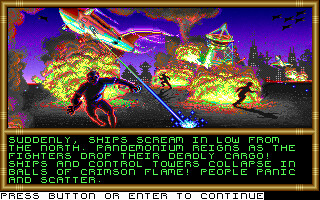This image is a screen capture from an old retro-style video game characterized by low-resolution graphics and a nostalgic aesthetic. The scene unfolds in a devastated city under a dark purple sky, where golden rocket ships, somewhat resembling aggressive alien invaders, unleash destruction. Explosions and crimson flames engulf the crumbling ships and control towers as frantic civilians scatter in panic. One of the ships is visibly firing a laser amidst swirling clouds of smoke. At the top right, five jets fly in formation, while a lone jet appears at the top left of the image. The action is framed by a light brown border, giving the appearance of a bamboo color. At the bottom, within a black box with green text, a paragraph sets the chaotic narrative: "Suddenly, ships scream in low from the north. Pandemonium rains as the fighters drop their deadly cargo. Ships and control towers collapse in balls of crimson flame. People panic and scatter. Press button or enter to continue." The entire scene conveys a sense of urgent calamity and apocalyptic destruction.